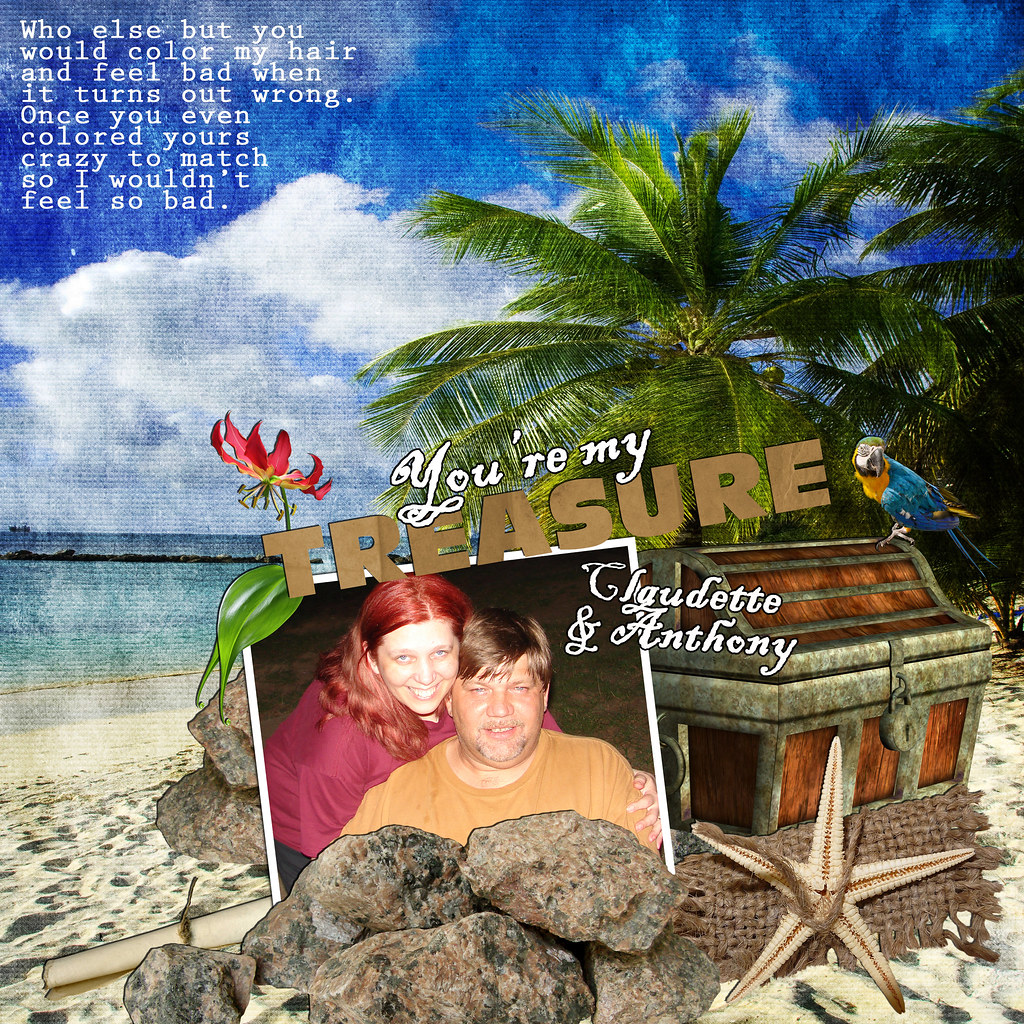The image showcases a picturesque beach scene with an ocean backdrop, featuring vibrant palm trees with lush green leaves. Central to the composition is an ornate treasure chest adorned with a colorful parrot, which has yellow chest feathers, a green head, a white face, and blue wings. In front of the chest rests a bright starfish. An inset photo depicts a smiling couple, Claudette and Anthony. Anthony, with short brown hair, is dressed in a yellow shirt, while Claudette, with red hair, wears a red shirt. Surrounding the couple's photo are various elements, including a pink and red rose, blending seamlessly into the scene. Above their photo, the text reads, "You're my treasure, Claudette and Anthony." In the top left corner, additional text states, "Who else but you would color my hair and feel bad when it turns out wrong? Once you even colored yours crazy to match so I wouldn't feel bad." The entire montage creates a heartwarming and visually engaging tribute.